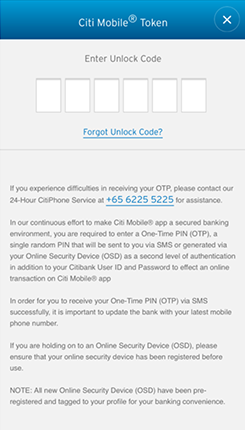A detailed caption for the given screenshot image could be:

"This image is a screenshot of the CITI Mobile app interface, featuring a tall and narrow layout with a blue banner at the top. The banner prominently displays the text 'CITI Mobile Token.' Below the banner, the interface prompts the user to 'Enter Unlock Code,' accompanied by three white squares for code input. Users are given the option to select 'Forgot Unlock Code?' for assistance.

Further down, the screenshot contains a detailed informational message. It explains that for enhanced security in the CITI Mobile app, users are required to enter a one-time PIN (OTP) for authentication. This OTP can be received either via SMS or generated through an Online Security Device (OSD). The message emphasizes the importance of updating the bank with the user's latest mobile phone number to successfully receive the OTP via SMS. It also mentions that new Online Security Devices (OSDs) are pre-registered and tagged to the user's profile for convenience.

For additional support, users are directed to contact CITI's 24-hour phone service at 1-800-625-5225. The image does not feature any people."